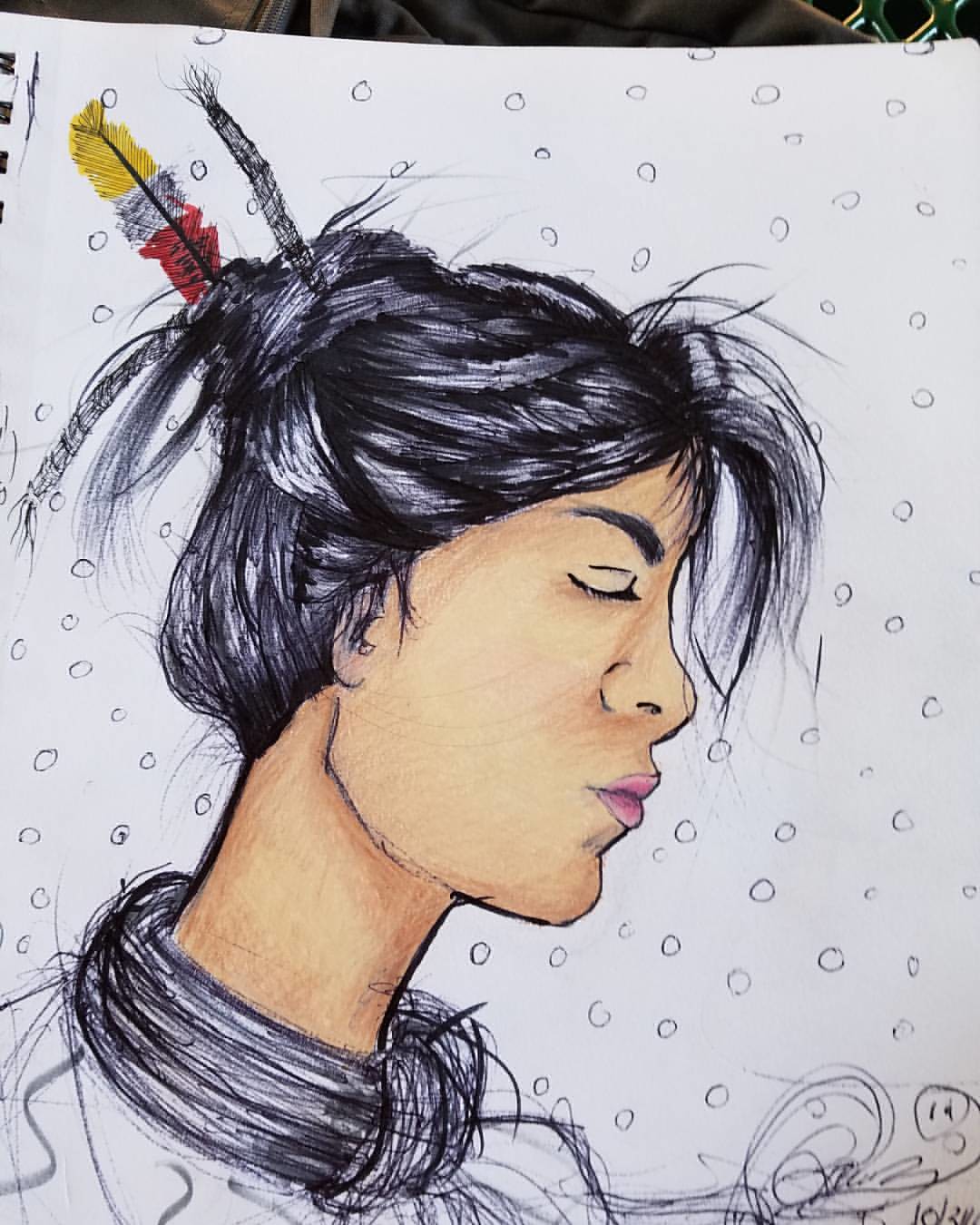This is a highly detailed pen and ink or pencil drawing of a Native American woman, rendered on white paper. The woman, who has a deep tan complexion, is shown in a side profile facing to her left, with her single visible eye gently closed. Her black hair is styled in a messy bun adorned with a prominent red, yellow, and white feather, accompanied by a few other dark-colored feathers. A few strands of her hair, including a noticeable droop of bangs, fall gracefully in front of her face. She is wearing a thick, intricately pencil-drawn collar, scarf, or necklace around her neck. Her lips are delicately colored in pink. The background features a pattern of small, round, open dots that enhance the overall composition of the image.